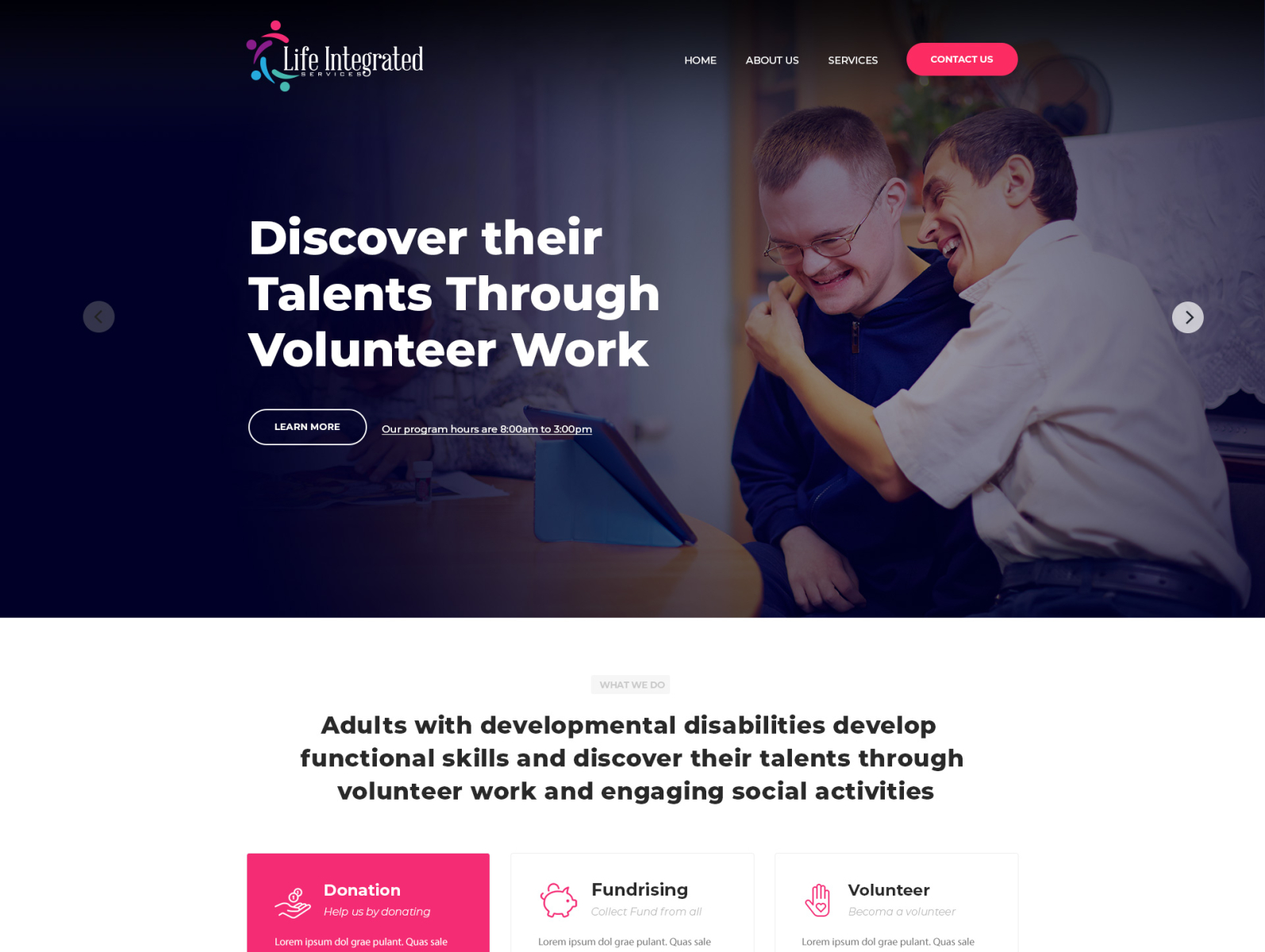A vibrant screenshot from the "Life Integrated" website featuring white lettering near the top identifying the site's name. To the left of the text, a logo displays artistic swirls in red, purple, and blue. Positioned on the right side, the navigation menu includes "Home," "About Us," "Services," and a prominent red "Contact Us" button with white text.

Just below, the main section showcases a heartfelt photograph of a man hugging an individual who appears to have a disability. To the left of this image, a call to action is displayed in white letters: "Discover their talents through volunteer work." Further down, additional information reads, "Learn more: Our program hours are 8 a.m. to 1 p.m." The section elaborates: "Adults with developmental disabilities develop functional skills and discover their talents through volunteer work and engaging social activities."

Beneath this informative segment, there are three rectangular boxes. The first features a red "Donation" button with white text. Adjacent to it, the second box is labeled "Fundraising" and includes an icon along with some descriptive text beneath it. The third box is titled "Volunteer," also accompanied by an icon and additional text.